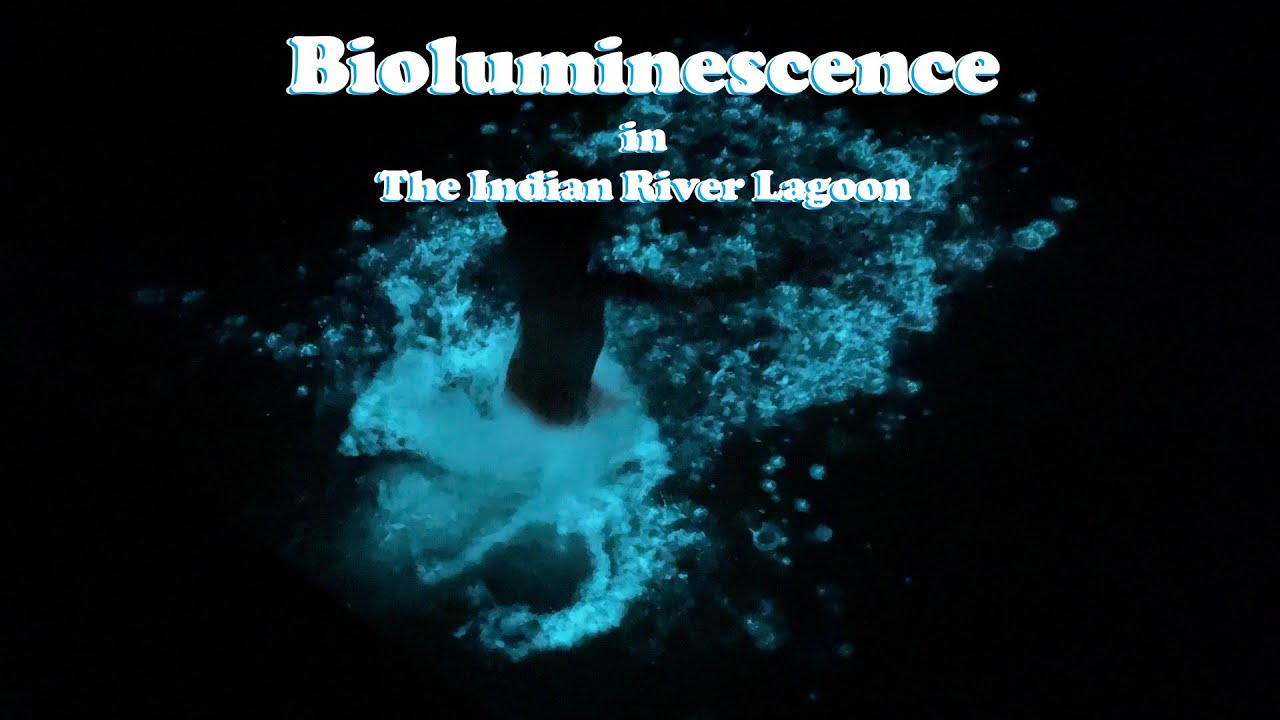In this image, we're presented with a movie-style design centered around a predominantly black background. At the very top of the image, in crisp white letters outlined with light blue, the word "B.I.O.L.U.M.I.N.E.S.C.E.N.C.E" is prominently displayed. Directly beneath it, in similar white and light blue typography, the text reads "IN" and then "The Indian River Lagoon". The area below these inscriptions features a texture reminiscent of light blue water patterns, giving a fluid and dynamic look. Dominating the central portion of the image is a large light blue shape from which a dark black silhouette emerges, adding a sense of mystery and intrigue. The stark contrast between the light elements and the black background emphasizes the title and central figure, creating an eye-catching visual that hints at an aquatic theme.